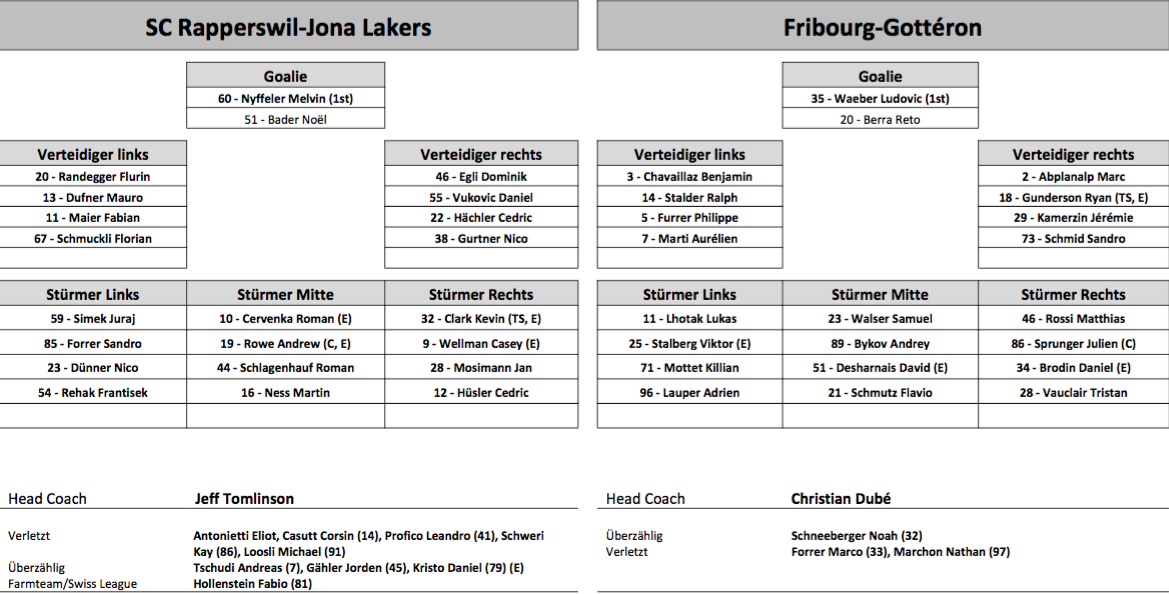The image depicts a black and white pregame printout for a sports match, featuring two teams. At the top, in gray and black letters, it reads "SC Rapperswill Jonah Lakers," accompanied by a detailed chart below that lists player positions with headings such as Goalie, Wertlinger Links, Wertlinger Rex, Sturmer Links, Sturmer Might, and Sturmer Rex. Adjacent to this chart is a similar grid titled "Freeburg Grotten," with identical column headings. Below each team's chart, the head coaches are named: Jeff Tomlinson for the SC Rapperswill Jonah Lakers and Christian Doob for the Freeburg Grotten. The entire layout is rectangular and dominates the overall image, which appears to be a simple printed sheet providing an overview of the teams and their player lineups. The image is devoid of any other objects or colors beyond black, white, and gray text.